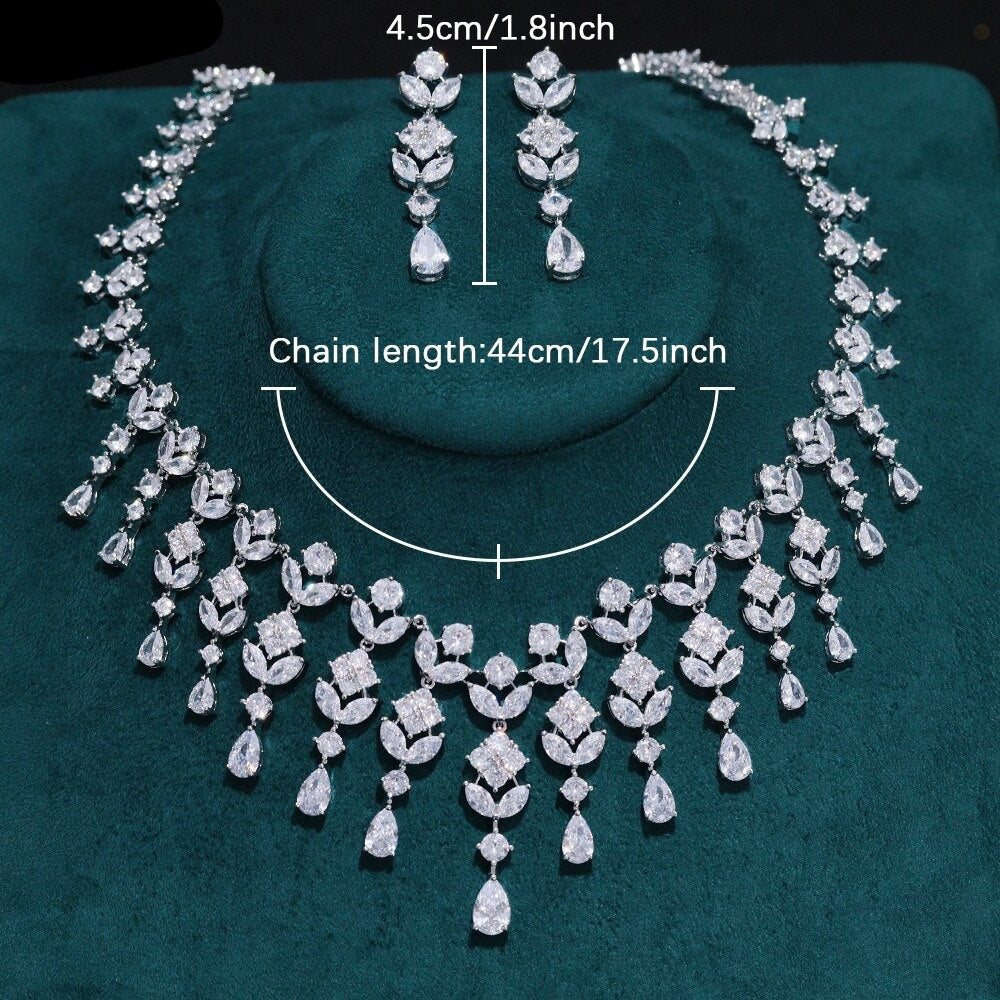The photograph showcases an elegant jewelry set displayed on an emerald faux suede bust. The display surface has a rounded and slightly raised section in the center, mimicking the neckline and shoulders. The background is black, which highlights the intricacy of the jewelry. The necklace, which forms a smooth curve around the bust, has a total chain length of 44 centimeters (17.5 inches). The chain is composed of repeating crystal-like pieces, each measuring 4.5 centimeters (1.8 inches). These pieces connect together and dangle gracefully, creating a visually captivating pattern. In addition to the necklace, a pair of earrings is prominently featured. These dangly earrings are laid out atop the circular raised section of the bust and consist of a series of circular, square, teardrop, and oval shapes, coordinating with the necklace's design. Text in white at the top of the image provides the measurements: "4.5 centimeters / 1.8 inches" for the earrings, and "chain length 44 centimeters / 17.5 inches" for the necklace. Overall, the image offers a detailed view of this sparkling and sophisticated jewelry set.